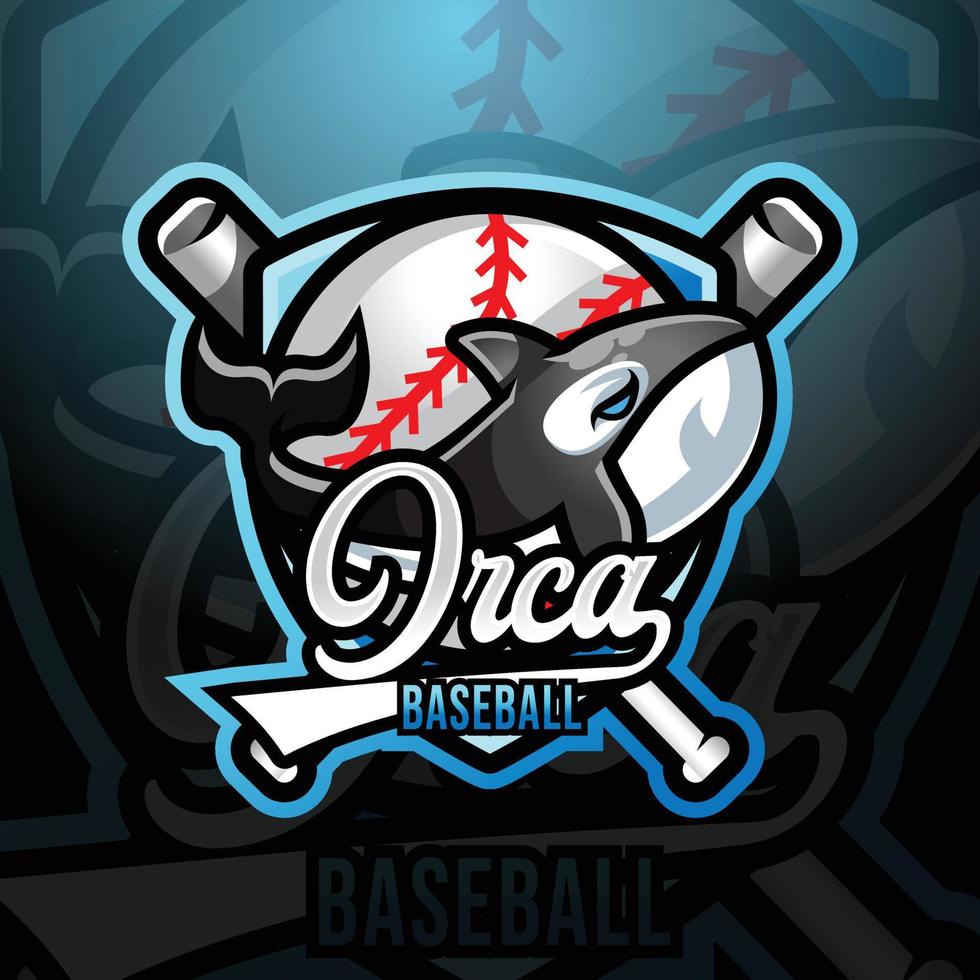The Orca Baseball team logo is a highly detailed and striking design that serves as both an advertisement and a visual emblem. At its core, the logo features a dynamic orca in different shades of black and dark gray, accentuated with a white underbelly and a vivid blue eye, swimming around a traditional white baseball with red cross-hatches. Two white baseball bats are crossed behind this central imagery, adding a classic touch. The text "Orca" is prominently displayed in a gradient from white to light gray in cursive, while "Baseball" sits just below it, rendered in a gradient from light blue to dark blue. The entire logo is color-coordinated with dark blue, black, light gray, and dark gray tones, contributing to its overall bold and sophisticated aesthetic. This logo is superimposed on a larger, transparent version of the same image, creating a sense of depth. The square-shaped poster, which could be seen in places like subway stations, is reminiscent of a decal or sticker, making it not only a functional promotional material but also a captivating piece of art for fans.